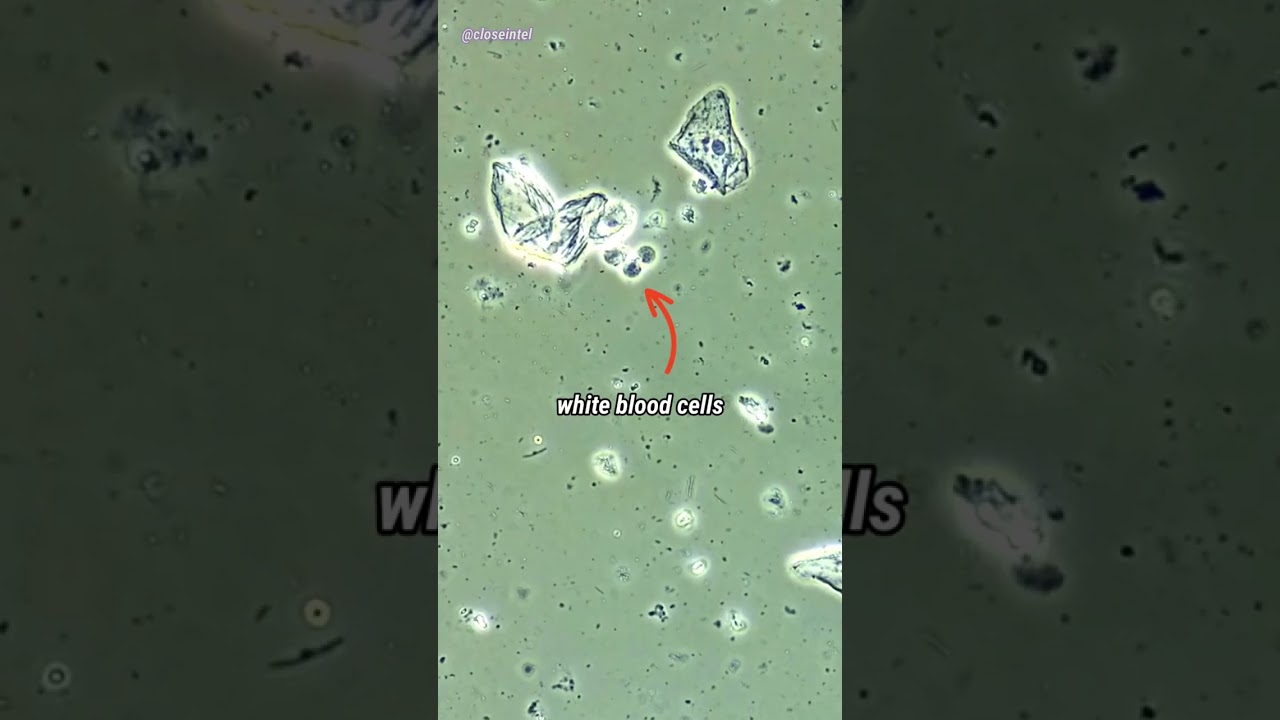The image is a detailed microscopic shot featuring white blood cells, set against a backdrop that appears to be a darker, more diffused version of itself. The central portion of the image occupies the vertical midsection, highlighted by a red arrow pointing to a larger, more complex white blood cell. The white cell is identifiable in part due to the text label "white blood cells" in small white font. Surrounding this central white blood cell are smaller, varied shapes and structures, possibly other cells or particles, some of which the white blood cell seems to be interacting with or consuming. The scene is set within what resembles a Petri dish environment. To the top left corner of the image, there is fine text reading "@closeintel," attributing the source or copyright. The visual effect includes a greenish, web-like background with scattered blue spots, enhancing the focus on cellular interactions within the sample.